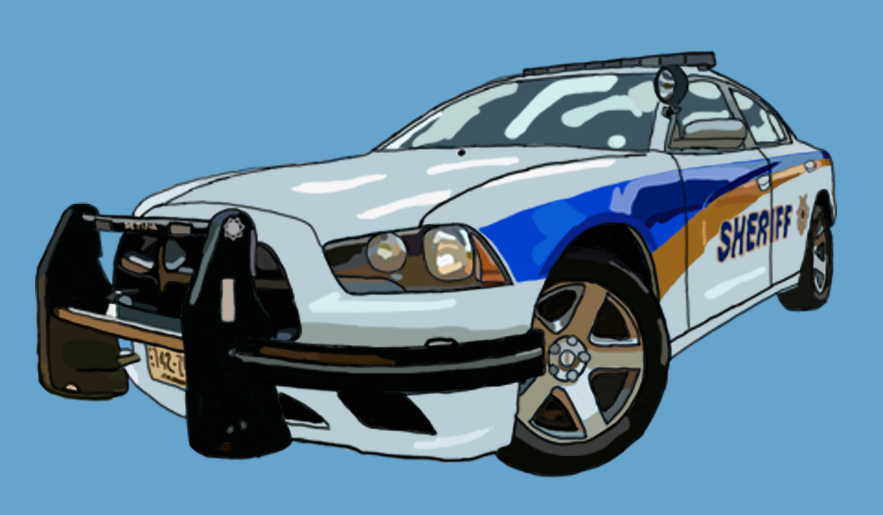An animated illustration of a sheriff's police car set against a sky blue background. The vehicle is predominantly white, featuring a prominent black grille at the front. The car's license plate reads "E142," positioned beneath a visible headlight on the left side. Running along the side of the car, a blue stripe is accented by a parallel yellow stripe. Bold blue lettering spells out "Sheriff," overlaid with a detailed badge icon. The car rests on sleek, black wheels and is equipped with a side mirror. Atop the vehicle, a large, unlit siren extends across almost the entire width of the roof. This detailed depiction captures the essence of a police car through its animated style, giving it a distinct, illustrative charm.